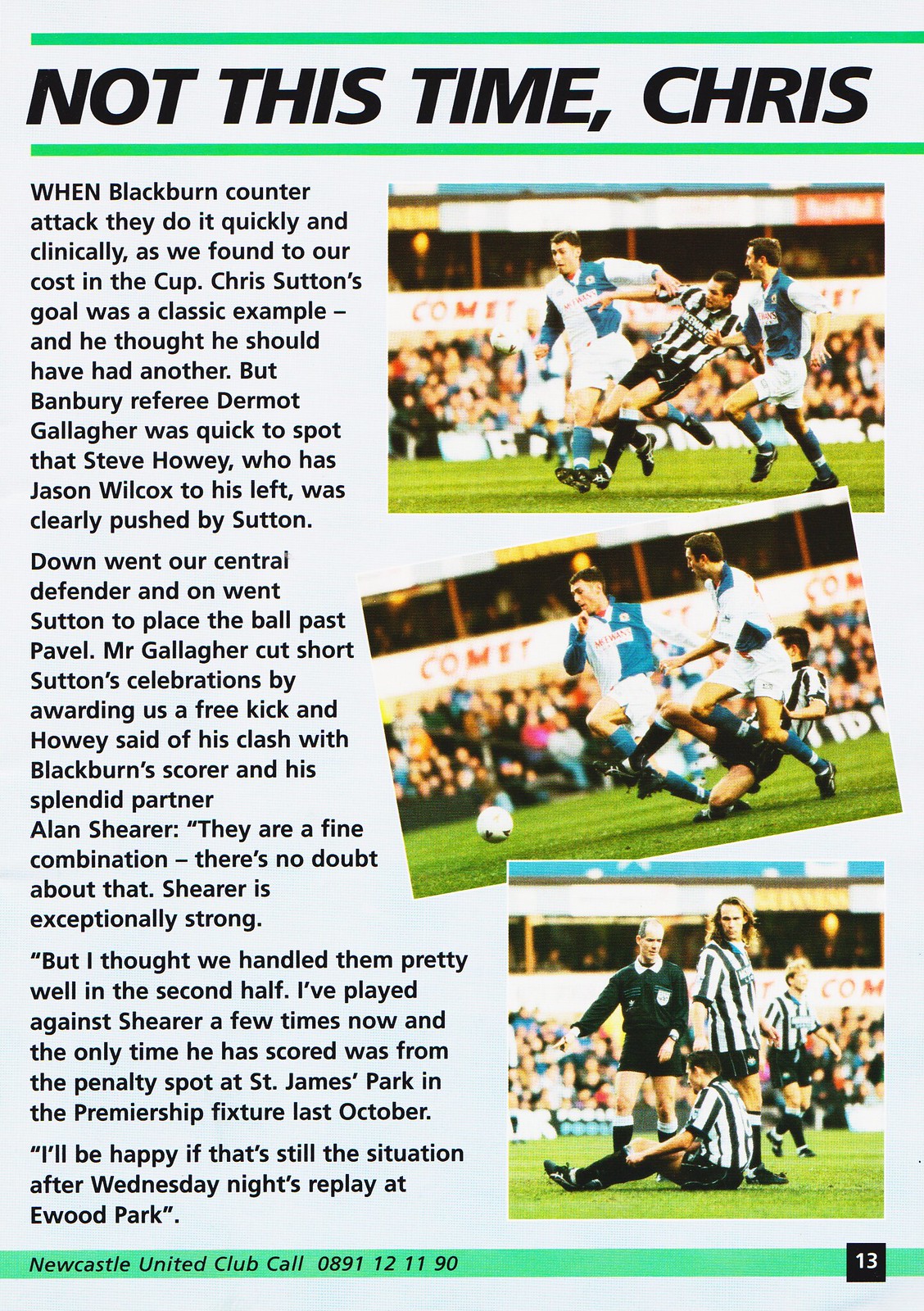The image is a tall rectangular flyer with a light grayish-blue background. At the top, framed by two bright green horizontal lines, the bold, italicized, all-capital black headline reads "NOT THIS TIME, CHRIS." On the right side of the flyer are three sequential photographs depicting a soccer match, showing a referee's fall. In the first image, a referee appears to stumble between two players, one in turquoise and another in white uniforms. The second photograph captures the referee closer to falling, while in the third, he is on the ground examining his knee. To the left of these images, there are three columns of text written in black font, providing a detailed commentary on the match. The bottom of the flyer features a thicker green rectangle with italicized black text reading "Newcastle United Club Call."